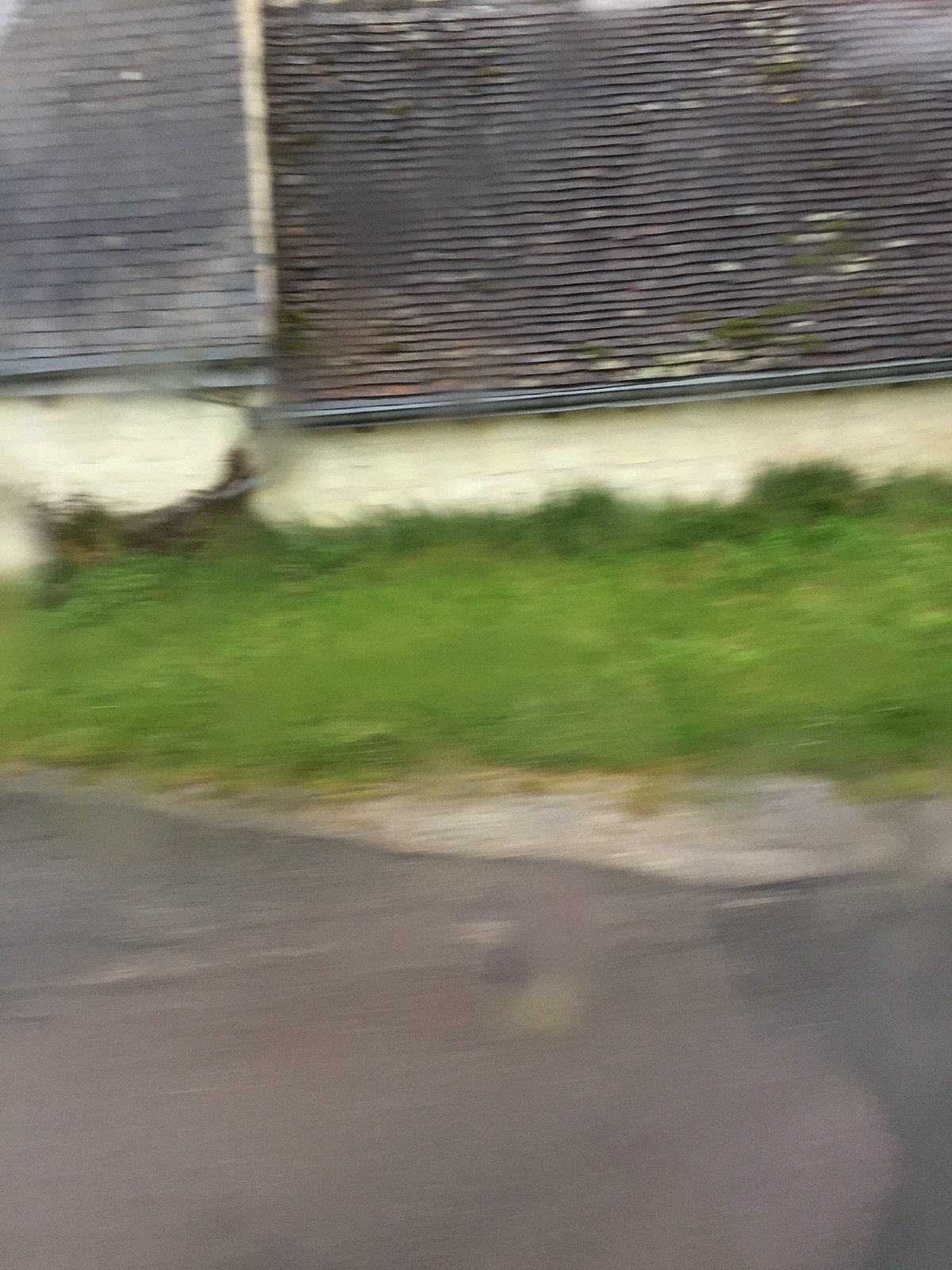A severely blurred photograph captures a colorful, though indistinct, outdoor scene. Dominating the center is a patch of green grass, framed below by what appears to be a gray road or sidewalk. Above the grass, a stretch of white brick interrupts the composition, leading to a gray area at the top, where either metal shingles or door shutters reside. The entire image suffers from extreme motion blur, making it seem as though the photo was taken mid-run, and transforming distinct elements into abstract swaths of color. Upon closer inspection, the gray section at the top is speckled with patches of moss or lichen, adding a touch of nature’s embellishment to the indistinct silver surface.